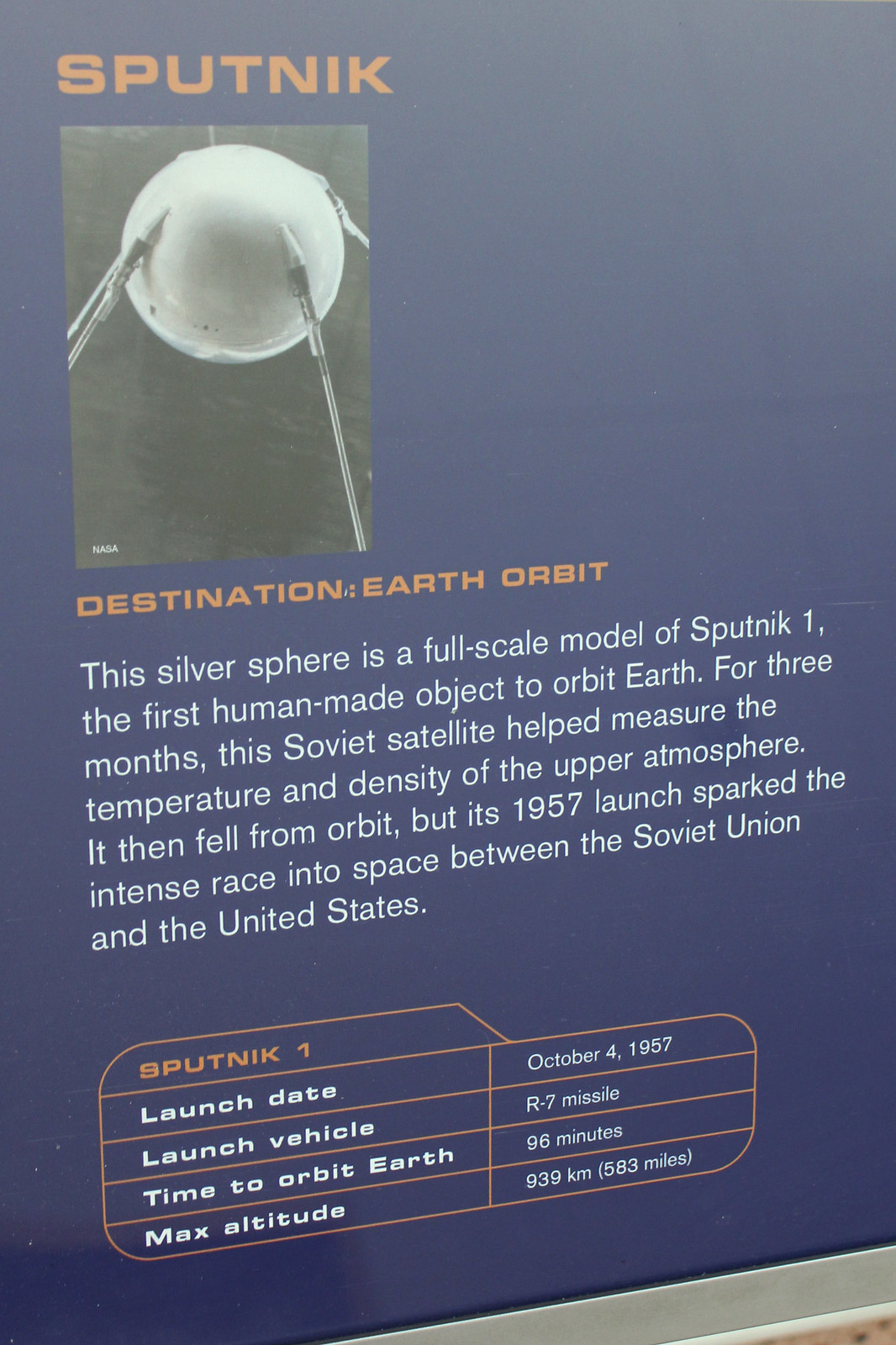The image displays a museum sign with a navy blue background. At the top left corner, it features the title "Sputnik" in orange. Beneath the title is a black and white photograph of a silver sphere, identified as a full-scale model of Sputnik 1, the first human-made object to orbit Earth. The subtitle, "Destination Earth Orbit," is also highlighted in orange. The sign includes a descriptive paragraph in white text that explains how, for three months, the Soviet satellite Sputnik 1 helped measure the temperature and density of the upper atmosphere before falling from orbit. Launched on October 4, 1957, by an R-7 missile, Sputnik’s journey, taking 96 minutes to orbit Earth and reaching a maximum altitude of 939 kilometers (583 miles), marked the beginning of the intense space race between the Soviet Union and the United States. At the bottom, an orange-chart format presents the satellite’s key data, including the launch date, launch vehicle, orbit time, and maximum altitude.